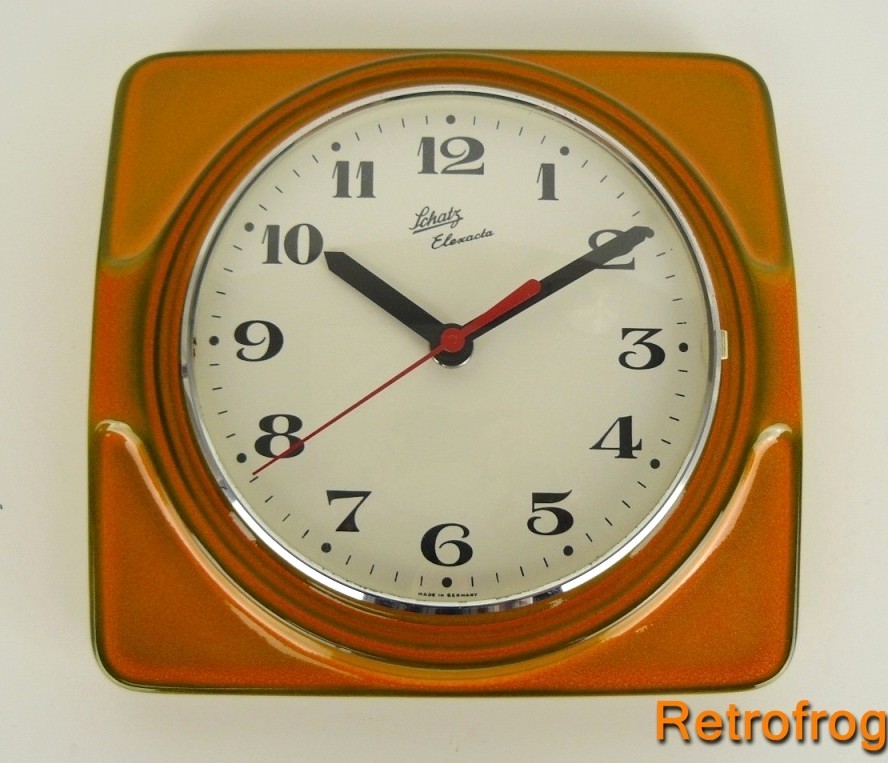This detailed photograph captures a vintage analog clock set against a neutral gray background. The clock, adorned in a plastic case of a warm amber-orange hue, exudes retro charm. Prominent at the lower right corner of the image is a watermark reading "Retro Frog" in vivid orange lettering, subtly attributing the image's origin.

Central to this nostalgic timepiece is a metallic silver ring encircling the clock face, lending a touch of elegance and contrast to the bold design. Adorned in black, the hour and minute hands gracefully sweep across the dial, punctuated by a vibrant red second hand that adds a dash of color and movement.

The face of the clock, branded with the name "Schatz Alexacta" at its core, features distinctive, stylized numerals reminiscent of an antique aesthetic. Each numeric hour is marked with sophisticated, vintage-inspired digits, while minute increments are indicated by slim, subtle slots. Dots further highlight each hour for added clarity and design coherence.

The clock's molded plastic casing is shaped into a square with gently rounded corners, enhancing its smooth, polished look. This piece harmoniously blends function with nostalgic style, making it a standout addition to any vintage decor enthusiast.